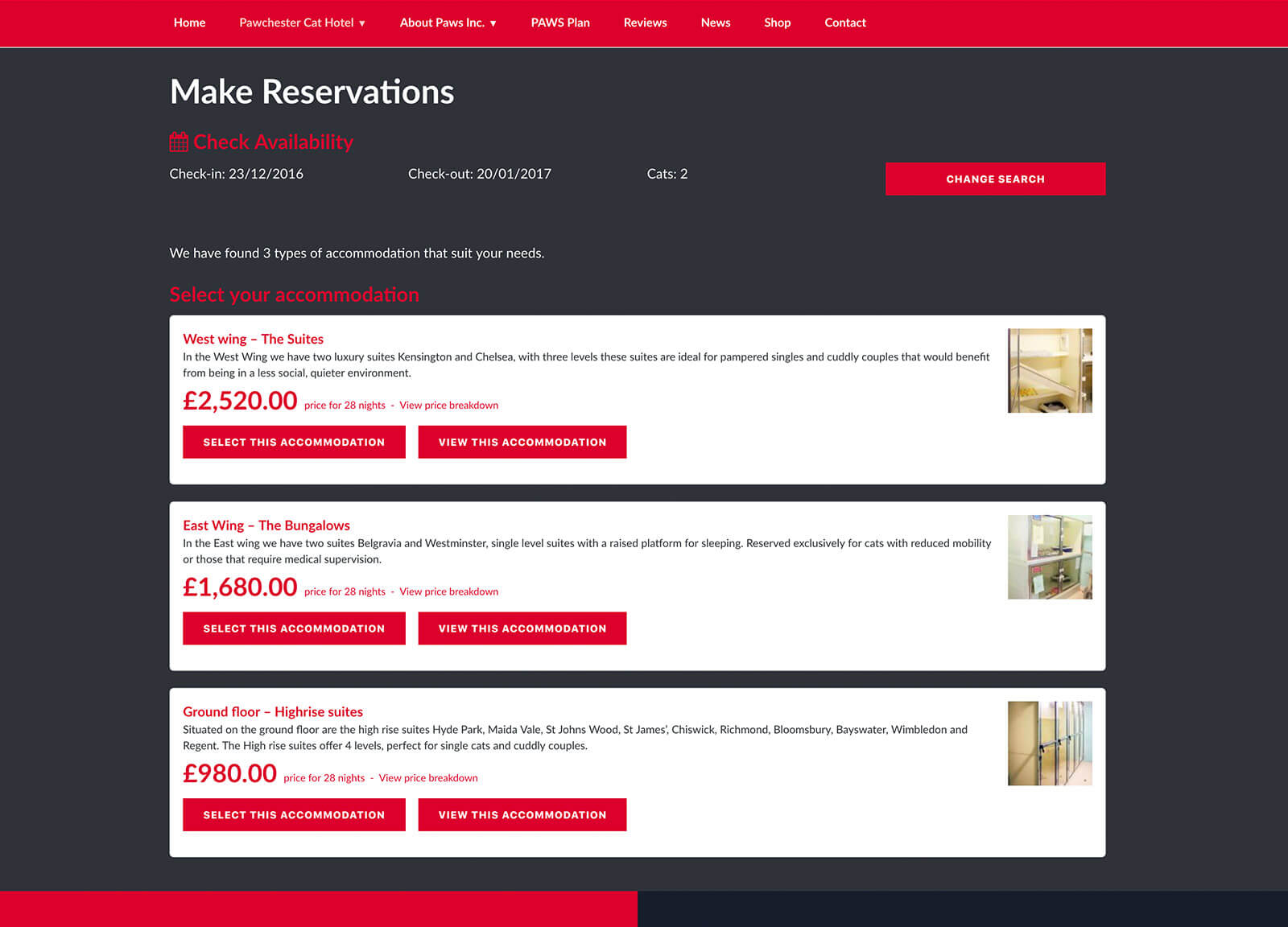The image depicts a pet-friendly hotel reservation page with a predominantly black background accentuated by red. At the very top of the webpage, there's a red menu bar with white text listing various options: Home, Paychester, Car, Hotel, About, About Paws Incorporated, Paws, Plans, Reviews, News, Shop, and Contact.

Beneath the menu bar, users have an option to make reservations by checking availability. The pre-selected dates shown are from December 23, 2016 (check-in) to January 20, 2017 (check-out), and the search is for one person with two cats.

The search results display three types of accommodations tailored to the user's needs:

1. **West Wing, The Suites**:
   - Price: $2,520 for 28 nights
   - Description: A brief description is provided.
   - Options: Users can select this accommodation or view more detailed information.
   - Image: There is an image showing part of a room, possibly a shelf.
   
2. **East Wing, The Bungalows**:
   - Price: $1,680 for 28 nights
   - Description: A brief description is provided.
   - Options: Users can select this accommodation or view more detailed information.
   - Image: Displays what appears to be a living room.

3. **Ground Floor, High Rise Suites**:
   - Price: $980 for 28 nights
   - Description: A brief description is provided.
   - Options: Users can select this accommodation or view more detailed information.
   - Image: Shows a community shower setting, though it is intended as an individual suite.

Each accommodation option is presented in a white bar with the key details and action links to either select or view the accommodation. The emphasis is on providing a clear choice for potential guests looking for pet-friendly stays.